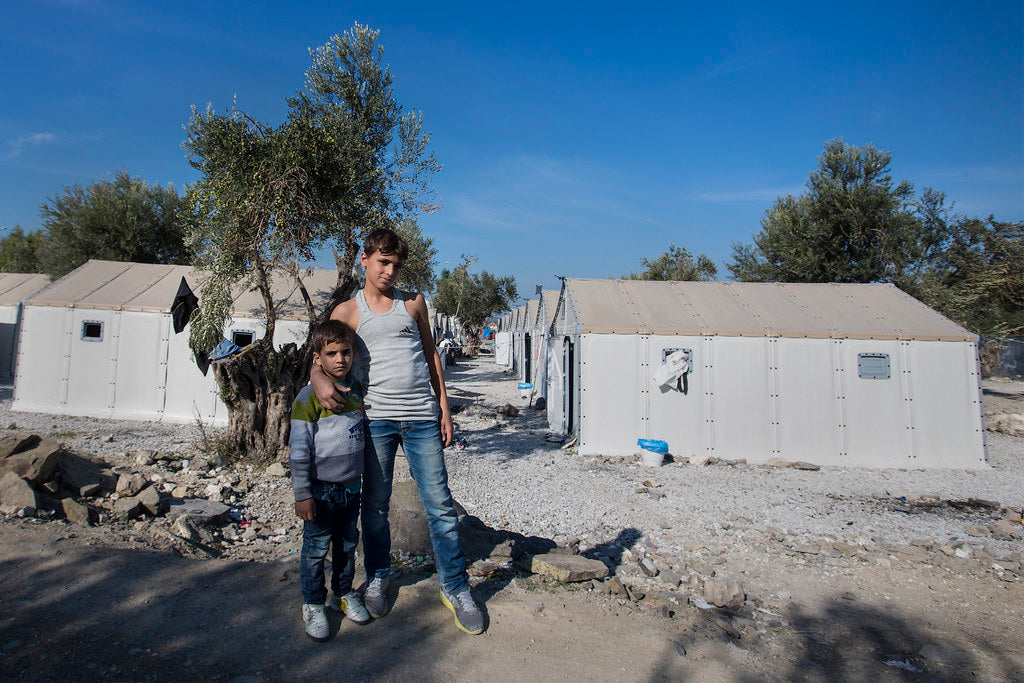In this image, a teenage boy stands to the right of a younger child, possibly his little brother, who appears to be around 5 or 6 years old. The older boy, with brown hair, is dressed in a gray, sleeveless Adidas tank top and blue jeans, along with gray tennis shoes. His arm is draped affectionately around the shoulders of the younger child. The younger boy is outfitted in blue jeans, white sneakers, and a white, green, and gray striped sweatshirt. They stand on a pale gray, rocky dirt road, which stretches behind them through a collection of rudimentary, metal-sided prefab buildings or tin sheds. Each structure features two windows, one normal-sized and the other smaller. The sheds extend in rows, suggesting it may be a residential area or work camp. In the background, trees with small leaves dot the scene, and a vibrant blue sky with a few clouds can be seen overhead. Additionally, a couple of white garbage cans with blue liners are placed outside the buildings. The boys pose for the picture, capturing a moment of camaraderie amidst a stark, utilitarian backdrop.